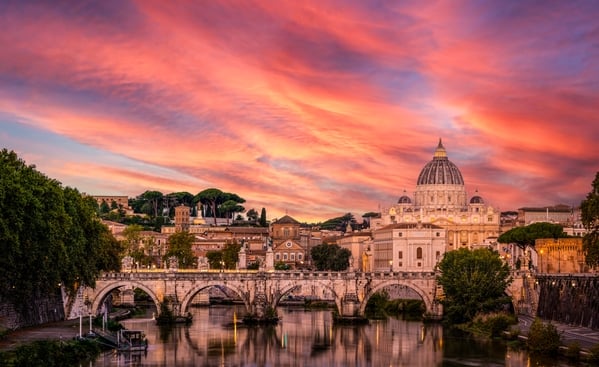The image depicts a detailed, picturesque painting of a European cityscape, likely a historic city like Rome. Dominating the scene is a grand, white building with a rotunda and a pointed top, evoking the architectural splendor of a capital building or important landmark. Adjacent to this building are closely packed, brownish concrete structures, some featuring domed roofs suggestive of churches or significant edifices.

A white bridge with four arches spans across a tranquil waterway in the foreground, reflecting parts of the city's architecture and lush greenery in its surface. A docked boat rests by the edge of the water, adding to the serene ambiance. Lining the waterway are trees, creating a touch of natural beauty amidst the urban setting.

The sky is particularly striking, taking up nearly half of the painting with its colorful display of blues, pinks, reds, and oranges, indicative of either dawn or dusk. This vibrant sky backdrop enhances the overall composition, casting an atmospheric glow over the city. The scene beautifully captures the blend of architectural grandeur and natural elements in this picturesque European city.